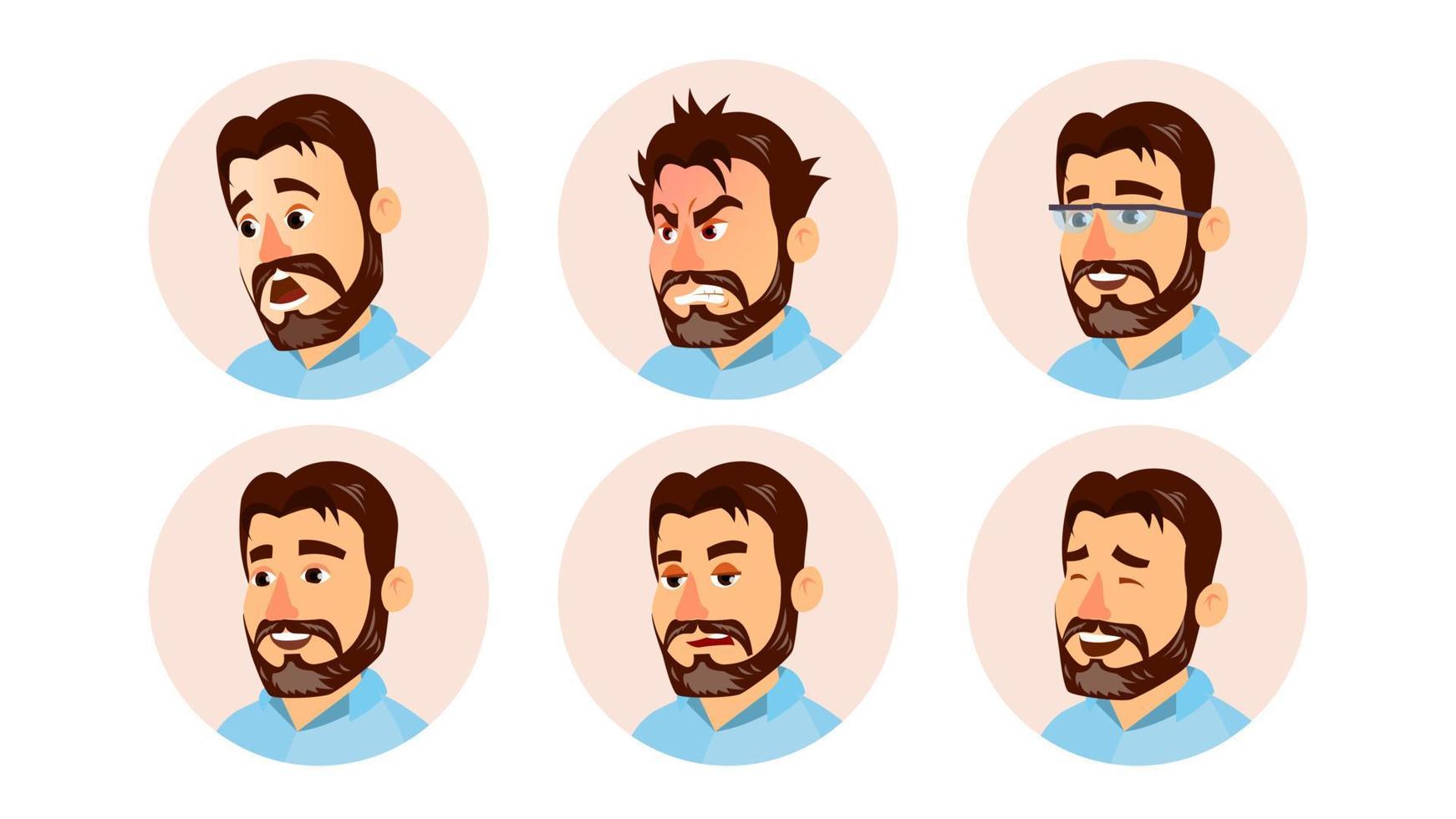The illustration features six different iterations of the same cartoon man, arranged in two rows of three. Each iteration is set within a beige circle. The man, a white individual with brown hair and a beard that wraps around his chin and connects to a mustache, has a lighter streak in his beard and highlights in his hair. His hair, which is parted in the center or slightly to his right, contains similar lighter accents. He has pale skin and a reddish nose. In each image, he wears a light blue collared shirt and is visible from the upper chest up, rendered in a classic Microsoft Illustrator black outline style.

The six images display a range of emotions: 
1. In the top left, he looks shocked and his gaze is directed downwards.
2. In the top middle, he appears very angry, with his face starting to turn red.
3. In the top right, he is happy, smiling, and wearing glasses.
4. In the bottom right, he is laughing, his eyes closed in amusement.
5. In the bottom middle, he has an uncertain expression with his mouth slightly open and his eyes somewhat closed.
6. In the bottom left, he looks cheerful and is smiling broadly.